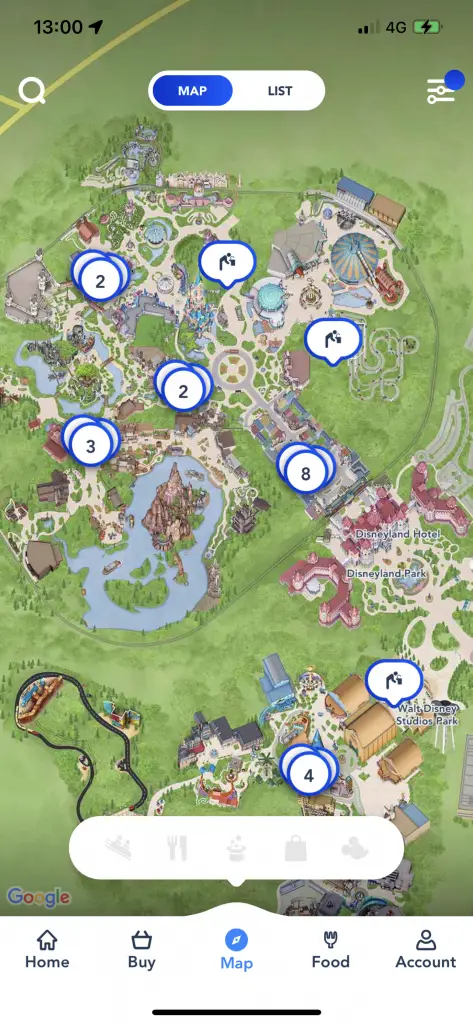The image depicts a detailed map from Walt Disney Studios Park, viewed on a smartphone. The phone displays a time of 13:00 in the top right corner, along with a signal strength of two bars and a 4G connection. The battery icon indicates a full charge. The map interface includes various elements: 

- Just beneath the time display is a white magnifying glass icon.
- Below that is a selection panel comprising a white oval with two options: "Map" and "List." "Map" is currently selected, highlighted with a blue oval and white text, while "List" remains in black.
- To the side is an icon featuring three lines with circles, likely indicating menu options for different map layers or features.

The map itself is largely green, indicating landscaped areas, with some brown patches representing pathways or buildings and blue regions denoting water bodies. Specific numbers such as 2, 2, 3, 8, and 4 mark various attractions or points of interest within the park. Additionally, there are icons signaling drink stations and other facilities.

Prominently labeled on the map are key locations like "Disneyland Park" and "Disney Hotel" to the right-hand side. Along the bottom of the map, several icons are displayed:

- A grayed-out roller coaster or log flume, symbolizing rides.
- A fork and knife, marking restaurants.
- A hat with stars, possibly indicating entertainment or shows.
- A shopping bag for retail spots.
- A mother and baby icon, likely pointing to restrooms with changing and feeding rooms.

Further below on the left side, the familiar Google logo appears in its trademark colors, followed by a navigation bar with icons and labels for Home (house icon), Buy (basket icon), Map (compass icon), Food (fork icon), and Account (person icon). 

This detail-rich map provides a comprehensive overview of Walt Disney Studios Park, aiding visitors in navigating the various attractions and amenities the park has to offer.